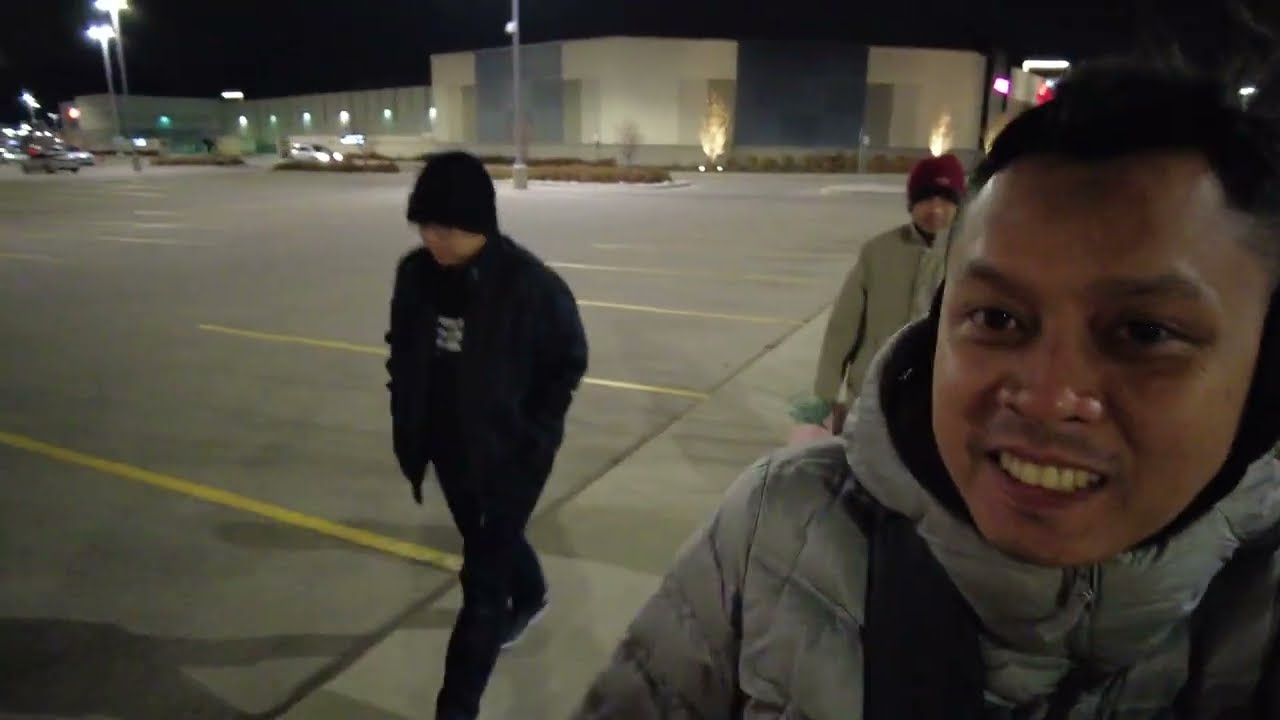The image captures a nighttime scene in an empty parking lot, illuminated by white street lights on silver poles, casting a glow over the area. The setting appears to be a school or a similar building, characterized by black or dark blue, tan, creamish, and greenish walls. There are a few cars in the distance, including a blurred silver van and a red car, lined up in yellow-painted parking spaces on a gray asphalt surface. Bushes and trees, some lit, adorn the scene. 

In the foreground, to the bottom right, are three men dressed warmly, suggesting it's winter. The man closest to the camera is smiling, seemingly taking a selfie. He is an Asian gentleman with short dark hair, wearing a puffy gray ski jacket and carrying a black backpack. To his left, another man clad in all black, including a beanie and a coat with white-bottomed sneakers, walks with his head down. His shirt has unreadable white text on it. Behind them, further back, is a man in a maroon beanie and a tan jacket, partially obscured and walking alongside them. The dark, starless sky serves as the backdrop, accentuating the scene's serene, nocturnal ambiance.